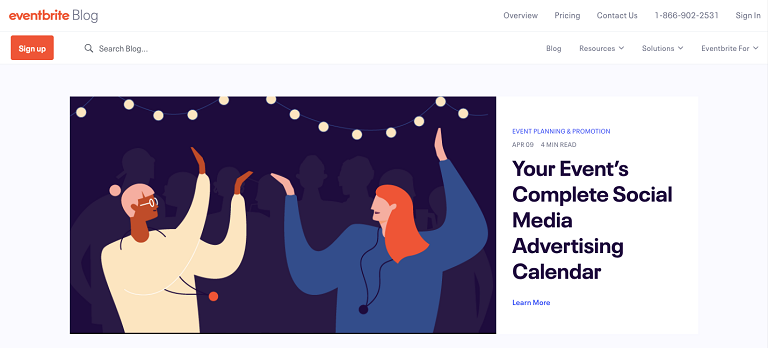This image is a screenshot from an Eventbrite blog page. In the top-left corner, the word "Blog" is displayed prominently. The navigation bar features drop-down menus for "Overview," "Pricing," and "Contact Us," along with a phone number, 1-866-902-2531, and a "Sign In" button. Directly below, to the left, is a red "Sign Up" button with white text, followed by a search bar for the blog, and additional drop-down menus for "Blog," "Resources," "Solutions," and "Eventbrite 4."

Central to the image is a colorful, cartoon-style illustration of two women with their arms raised. The first woman has tannish pink hair, wears white glasses, a yellow shirt, and a necklace with a red pendant. The background features string lights and silhouettes of people dancing. The second woman, who has orange hair, dons a blue shirt and a black necklace. To the side, the text reads, "Your Events Complete Social Media Advertising Calendar."